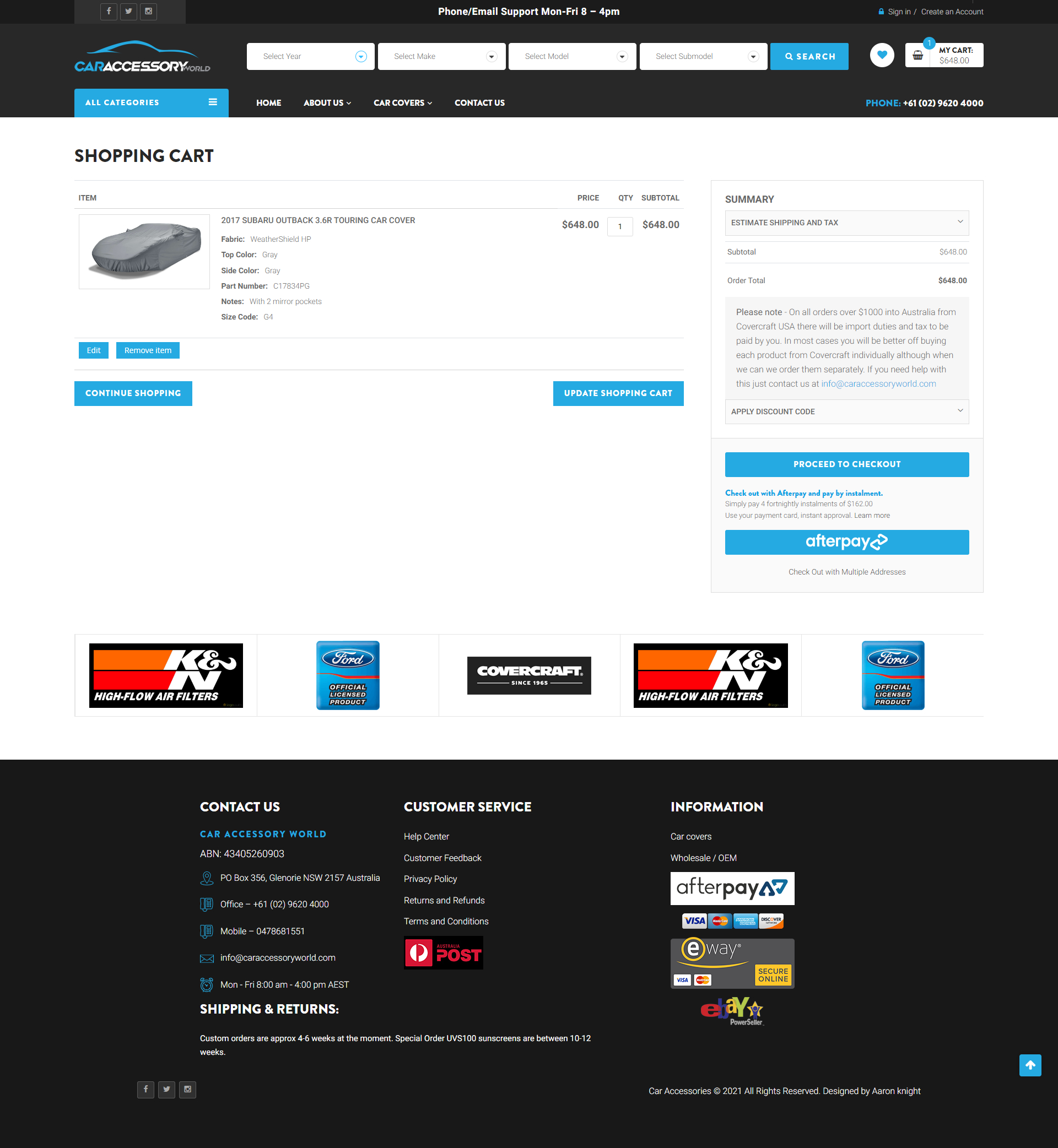The image appears to be a comprehensive screenshot of a webpage from a car accessory retail website named "Car Accessory World." In the top left corner, the website's logo and name are prominently displayed. Below, there are interactive dropdown fields labeled "Select Year," "Select Make," "Select Model," and "Select Sub-Model," accompanied by a blue "Search" button. In the upper right corner, an icon of a shopping cart provides access to the user's cart, indicated below with the text "Shopping Cart."

The shopping cart section displays a thumbnail image of a car covered with a gray cover, alongside a detailed product description: "2017 Subaru Outback 3.6R Touring Car Cover." The item is priced at $648. The quantity is set to one. Beneath this section are two buttons for further action: one blue button labeled "Continue Shopping" and another labeled "Update Shopping Cart."

On the right side, there's a summary box with the breakdown of costs, showing a "Subtotal" of $648 and an "Order Total" of $648. Directly below this summary is the "Proceed to Checkout" button.

Further down the page, there are colorful brand images with names such as "K&N High-Flow Air Filters," "Ford Official Licensed Product," and "Covercraft since 1965." At the very bottom of the page, a black rectangle contains company information, including a "Contact Us" section with phone numbers, addresses, a "Customer Service" link, and additional information.